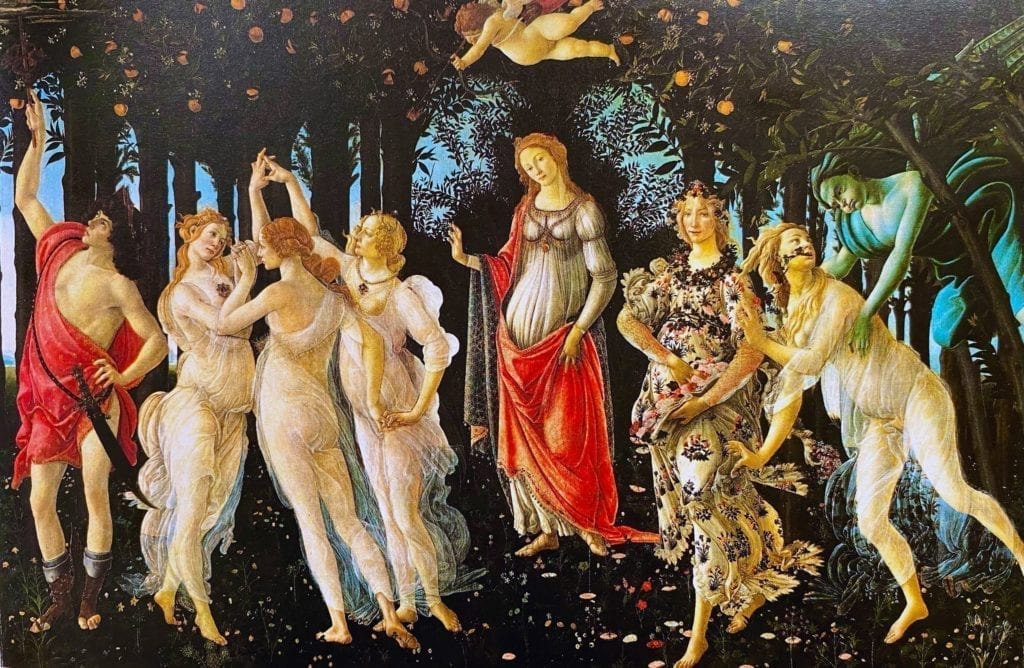This Renaissance painting portrays a mythological scene set in a dark, eerie forest or fruit grove. Central to the image is a woman wearing a grayish dress with a reddish overcoat, holding it at her waist. To her right, a bluish, ghostly figure is grabbing a woman who appears alarmed, while another woman, possibly pregnant, stands nearby. A little cupid hovers above the central figure, aiming an arrow. To her left, three women are dancing or frolicking, holding hands in a circular formation, and wearing transparent, sheer dresses. A male figure in a reddish robe stands among them, reaching for fruits in a tree. The background is densely forested with dark, muted colors, characteristic of Renaissance art. The sky is barely visible, adding to the mysterious ambiance.